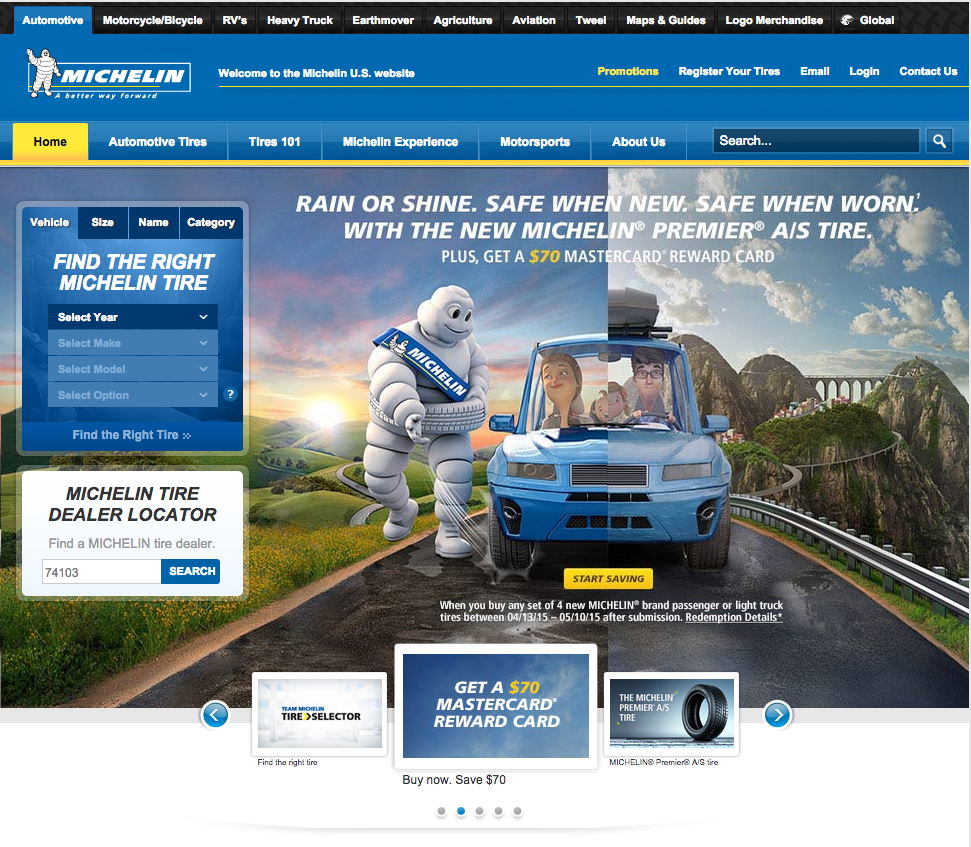Homepage of the Michelin Website

The featured image showcases the homepage of the Michelin website, renowned for its tires. The homepage is easily identifiable by the highlighted 'Home' category in yellow, setting it apart from the adjacent blue categories like 'Automotive'. A prominent Michelin logo, accompanied by the iconic Michelin Man, occupies the top left corner.

Navigation options are clearly laid out across the top, starting with the 'Automotive' section, followed by categories such as 'Motorcycle & Bicycle,' 'RVs,' 'Earthmover,' 'Aviation,' 'Maps & Guides,' 'Logo Merchandise,' and 'Global.' Below this navigation bar, a yellow button catches the eye with a call to action for promotions. Other options in this row include 'Register Your Tire,' 'Email,' 'Log In,' and 'Contact Us.'

The main content area prominently features the Michelin Man, depicted in his classic all-white attire and sporting a sash across his torso, reminiscent of a traditional gunslinger. He stands opposite a blue car filled with a family - parents and possibly two children - creating a warm, inviting atmosphere.

To the left of this scene is a functional search box offering various methods to find the right Michelin tire. Users can search by vehicle, tire size, name, or category. The example shown has 'Vehicle Search' selected, prompting users to input the year, make, model, and specific options of their vehicle. Below this, a white box allows users to find a Michelin tire dealer by entering their zip code.

At the bottom of the image, several promotional widgets are displayed. One offers a $70 Mastercard reward card, featuring arrows on either side to navigate through additional Michelin advertisements and deals.

Overall, the homepage is designed for easy navigation and quick access to essential information, ensuring users can find the products and support they need effortlessly.